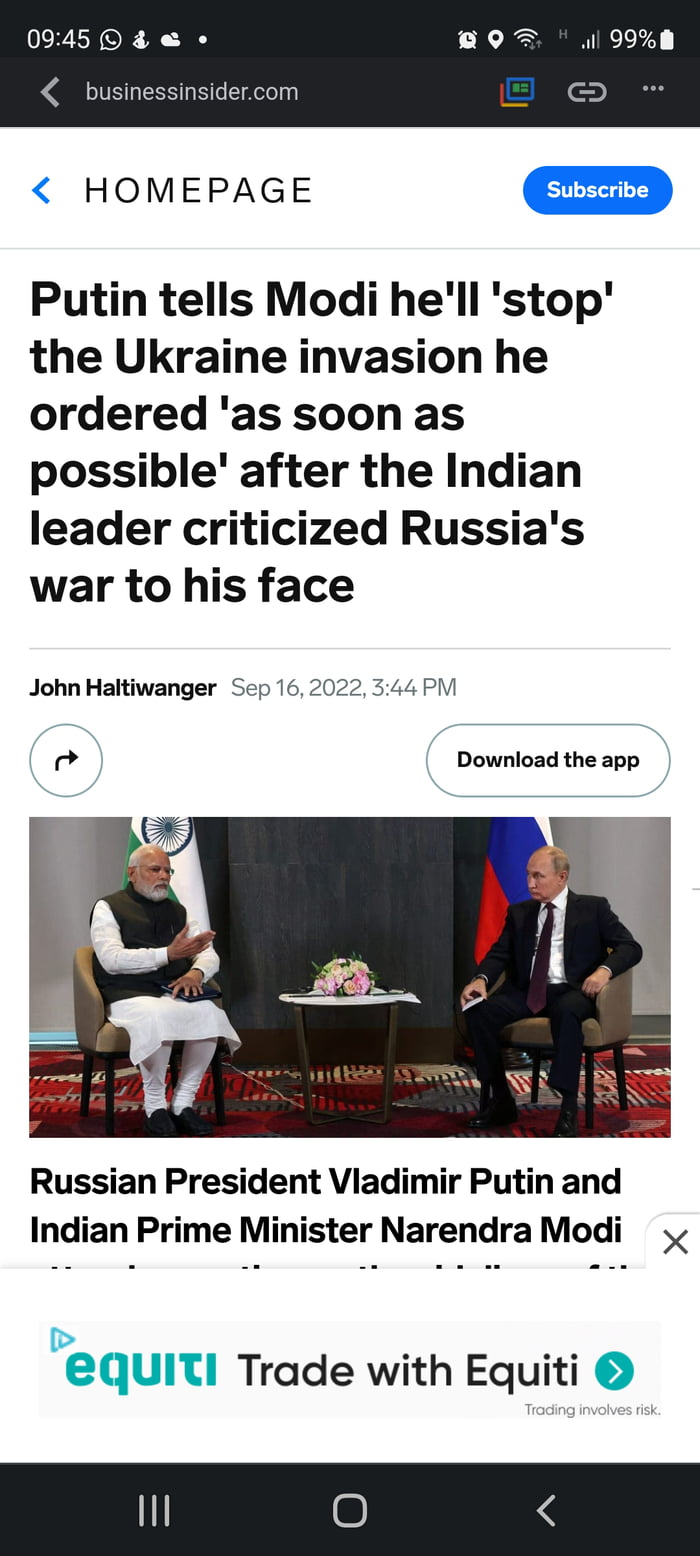This image is a screenshot of a phone display that captures a newspaper article. The screenshot, oriented in portrait mode, is significantly taller than it is wide. The photo is detailed and legible, despite some text appearing slightly compressed.

At the very top, a black rectangular notification bar spans horizontally across the screen, displaying the time (9:45), a WhatsApp chat bubble, and two unidentified icons, followed by an ellipsis indicating additional notifications. To the right, there's a series of icons: an alarm clock, navigation button, location button, WiFi signal, cellular network signal, and a battery icon showing 99% battery life.

Below the notification bar, the interface indicates "homepage" in grey font, accompanied by a blue leftward-facing arrow and a blue "subscribe" button to the far right.

The headline of the article reads: "Putin tells Modi he will stop the Ukraine invasion he ordered as soon as possible after the Indian leader criticized Russia's war to his face." The article is authored by John Halter Wenger and dated September 16, 2022, at 3:44 PM.

Directly below the headline is an image depicting Russian President Vladimir Putin and Indian Prime Minister Narendra Modi seated and engaged in discussion. Underneath the image, a subheader begins with "Russian President Vladimir Putin" and "Indian Prime Minister Narendra Modi" but is abruptly cut off by an advertisement banner at the bottom of the screenshot.